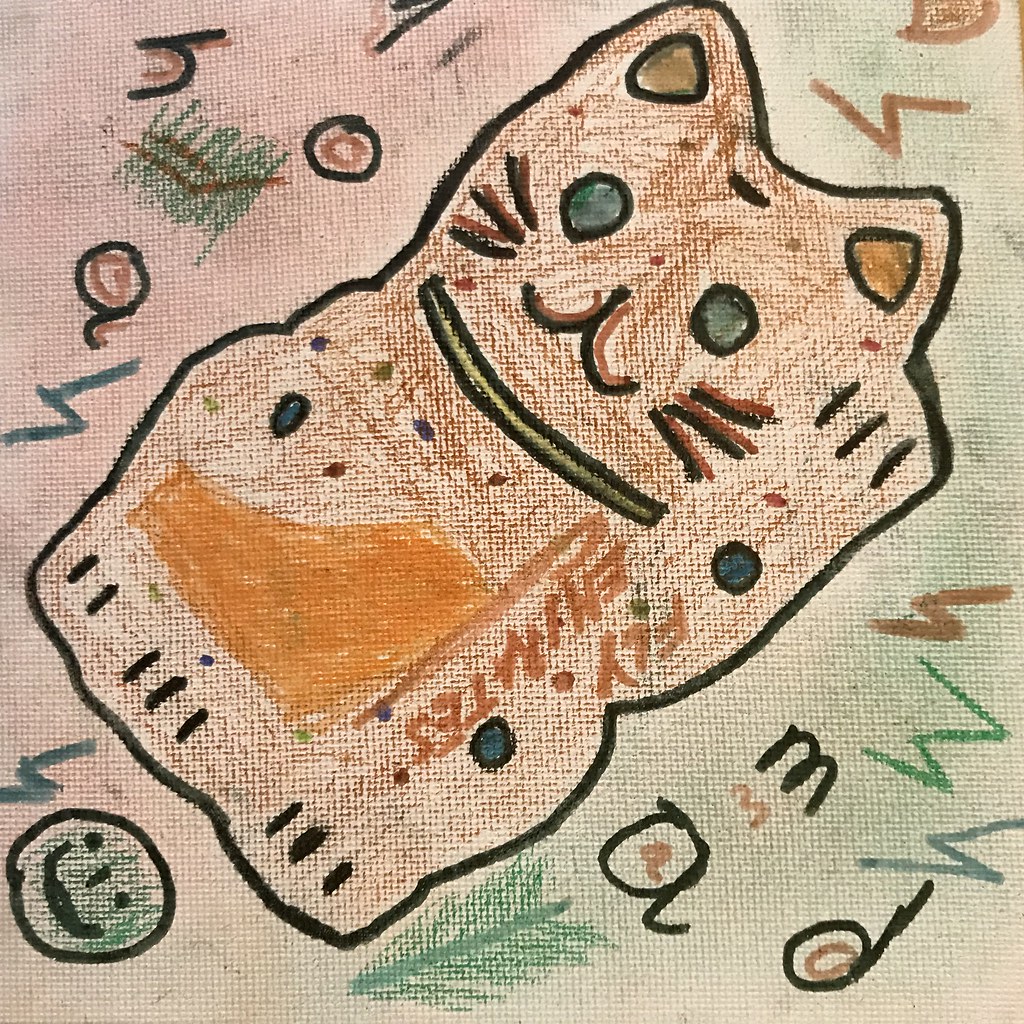The image appears to be a colorful drawing, likely crafted by a young child, combining crayon and marker. The background is a vibrant pink, adorned with overlapping letters in black and light brown. These letters—H, N, O, A, M, A, and D—are outlined twice, creating a layered effect. In the center, there's a rudimentary depiction of a cat with a square body but prominent ears. The feline features blue eyes, visible whiskers, and a simple smiley face. Scattered across the drawing are zigzag patterns reminiscent of lightning bolts. Additionally, the phrase "fly something" is written, although part of the text is illegible due to being upside down.